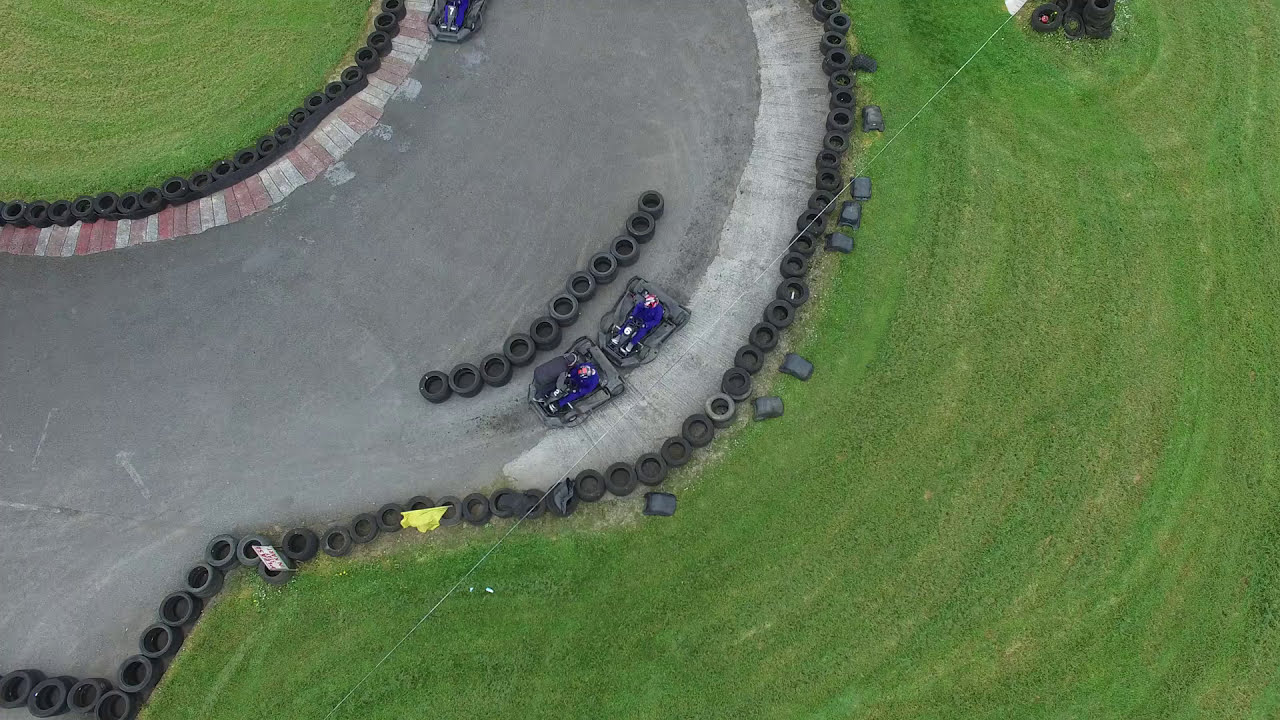The image captures an aerial view, likely taken from a drone, showcasing a go-kart track surrounded by well-maintained green grass, which appears freshly cut due to visible mowing lines. The cemented track is bordered by black tires for safety, ensuring racers remain within the designated area. On the track, there are three go-karts, two of which are closely positioned, with one touching the rear of the other, and the third partially visible in the top left corner of the image. The drivers, identifiable by their blue jumpsuits and red and black helmets, are seated in black-colored go-karts, suggesting a race setting. Additionally, two individuals are either sitting or laying down near what appears to be rubber mats or wraps, adding to the scene's dynamic nature. The bright daylight enhances the clarity and vividness of the entire scene.